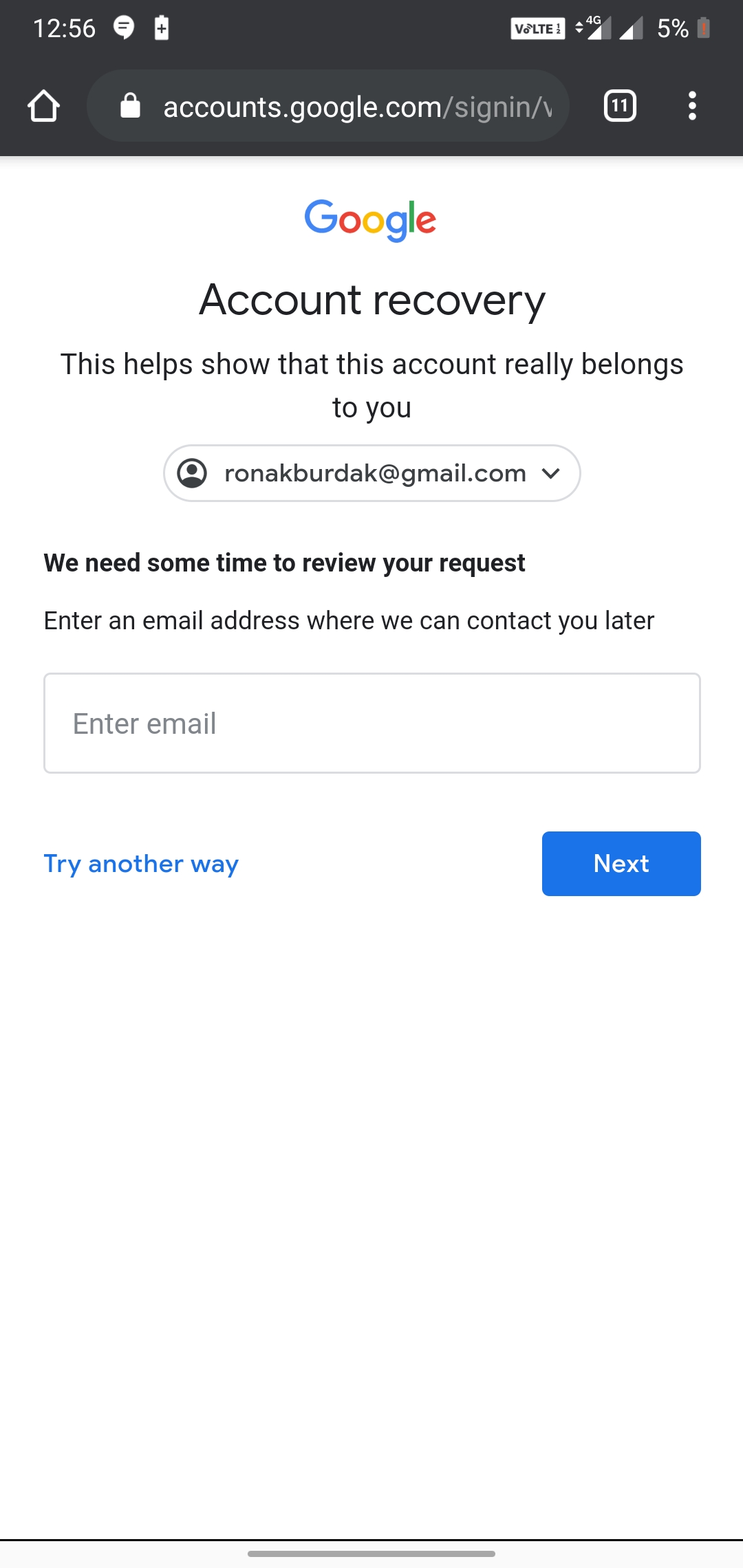The image is a vertically oriented rectangular screenshot taken from a cell phone. The upper portion of the image features a black horizontal banner displaying the time and various status icons, including a battery indicator showing a critically low charge at 5%. Centered within the banner is the web address "accounts.google.com," indicating it is a sign-in page for Google accounts.

Beneath the banner, the remainder of the screen has a white background. Prominently placed in the center is the colorful Google logo. Directly below the logo, the text reads "Account Recovery," accompanied by a message that states, "This helps show that this account really belongs to you." A drop-down menu follows, allowing the selection of the appropriate email address.

Further down, the instructions continue with "We need some time to review your request. Enter an email address where we can contact you later," followed by a field to enter the email address. Approximately in the center of the image, on the left side and in blue text, is a link labeled "Try another way." On the right side, positioned as a button, is the "Next" option for the user to proceed after entering their email address.

The bottom half of the screenshot is completely empty, showcasing no further text or icons.